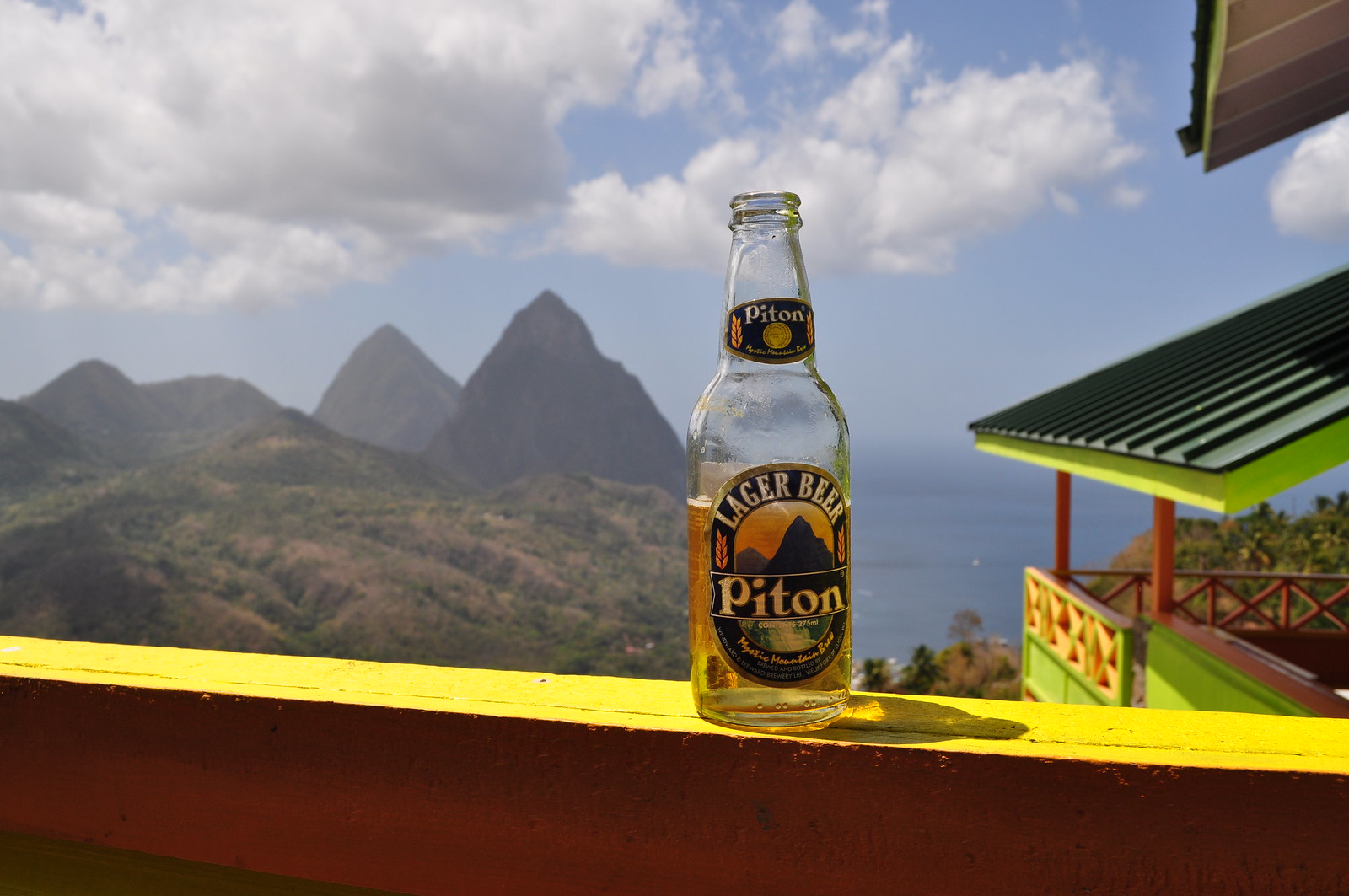The photograph captures a clear glass bottle of Pinon Lager Beer centrally positioned on a uniquely painted railing, with a vibrant orange base and yellow top. The bottle features two labels: an oval one on the main body and a smaller one around the neck. Both labels showcase yellow wheat sheaves, a black frame, and distinct white text—'Lager Beer' on the body label and 'Pinon' on both. The scenic background reveals a light blue sky adorned with white and light gray clouds, suggesting daytime. To the right, a vast blue body of water stretches out, while the left side is dominated by a series of mountain peaks, creating a picturesque setting reminiscent of the label's design, implying a restaurant terrace overlooking this stunning view.